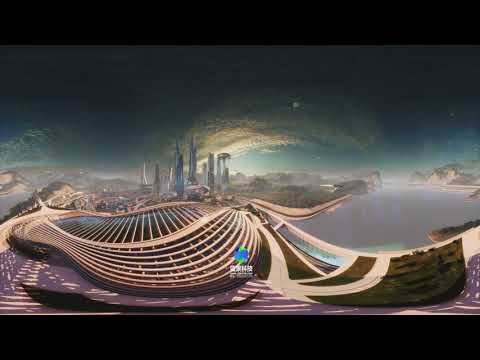The image appears to depict a futuristic cityscape, viewed from a considerable distance, perhaps through a digital or AI-generated filter, as suggested by its pixelation and slight blurriness. The scene features a sprawling skyline with numerous tall skyscrapers positioned predominantly on the left-hand side. A vast body of water, likely a lake, bordered by trees and grassy areas with walking paths, lies on the right-hand side. Within the water, there are large cliff faces providing a natural contrast to the urban environment. The foreground shows an intricate grid of iron beams and an expansive road or transit network, adding to the city's modern aesthetic. The upper portion of the image is dark with overcast clouds, giving it a night-time or twilight atmosphere, despite a faint hint of blue in the sky. Black borders frame the top and bottom of the image, reinforcing the sense of an artistic or digital manipulation.